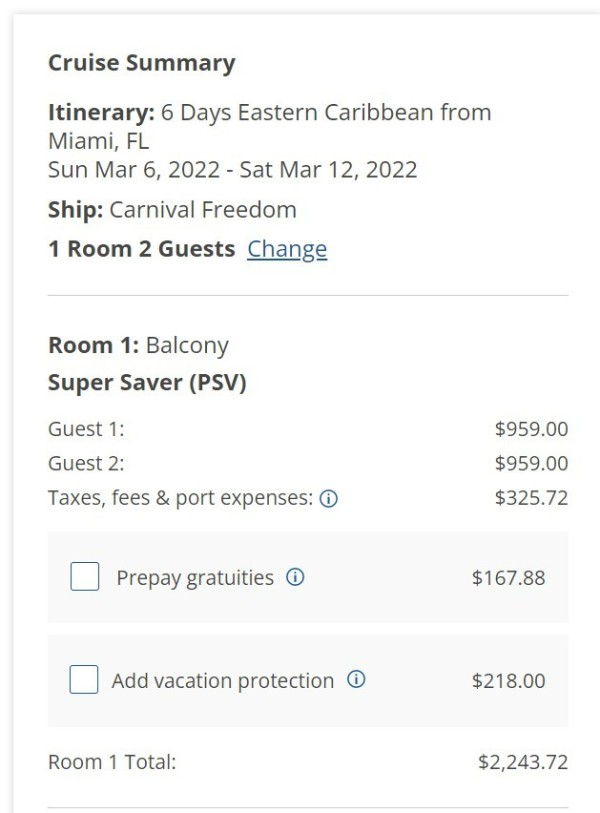The image depicts a detailed online booking summary for a cruise, arranged in a structured format on a predominantly white background, featuring left and top gray borders.

### Upper Section:
- **Title (Upper Left):** 
  - "Cruise Summary" in bold black font, left-justified.
  
- **Subtitle (Below Title):**
  - **Itinerary:** "Itinerary: 6 days Eastern Caribbean from" in bold black font followed by "6 days Eastern Caribbean" in non-bold font.
  - **Departure:** "Miami, FL" on a new line, left-justified and aligned below "Cruise Summary".
  - **Dates:** Initial-capped "Sun, Mar 6, 2022 - Sat, Mar 12, 2022," aligned with the aforementioned text.

### Middle Section:
- **Ship Information:**
  - **Ship:** "Ship: Carnival Freedom" in bold black font.
  - **Accommodation:** "One room, two guests" in bold black font. To the right, "Change" in blue, underlined as a clickable link.

- **Divider:** 
  - Thin gray line running horizontally, not extending to the edges, with empty space above and below.

### Fare Details:
- **Room Types:**
  - **Room 1:** "Room 1: Balcony" in bold followed by non-bold "Balcony."
  - **Rate:** Bold "Super Saver (PSV)" beneath "Room 1".

- **Cost Breakdown (Aligned to the Far Right):**
  - **Guest 1:** "$959.00," right-aligned.
  - **Guest 2:** "$959.00," right-aligned and aligned with Guest 1’s price.
  - **Taxes, Fees, and Port Expenses:** "$325.72" with a blue informational icon to its left, right-aligned with the previous prices.

- **Additional Options (Within Light Gray Rectangles):**
  - **Checkboxes (Unchecked):**
    - **Prepaid Gratuities**: "$167.88" to the right of an unchecked box, aligned horizontally.
    - **Add Vacation Protection:** "$218.00" beside another unchecked box, aligned horizontally with the text.

### Lower Section:
- **Total Cost:**
  - **Room 1 Total:** "$2,243.72" in non-bold text, right-aligned with the Guest prices above.

- **Bottom Border:**
  - Long gray underline extending nearly across the width of the image, providing a concluding visual boundary.

This detailed and neatly aligned layout ensures that all essential information, such as the cruise itinerary, accommodation details, and associated costs, are clearly presented.